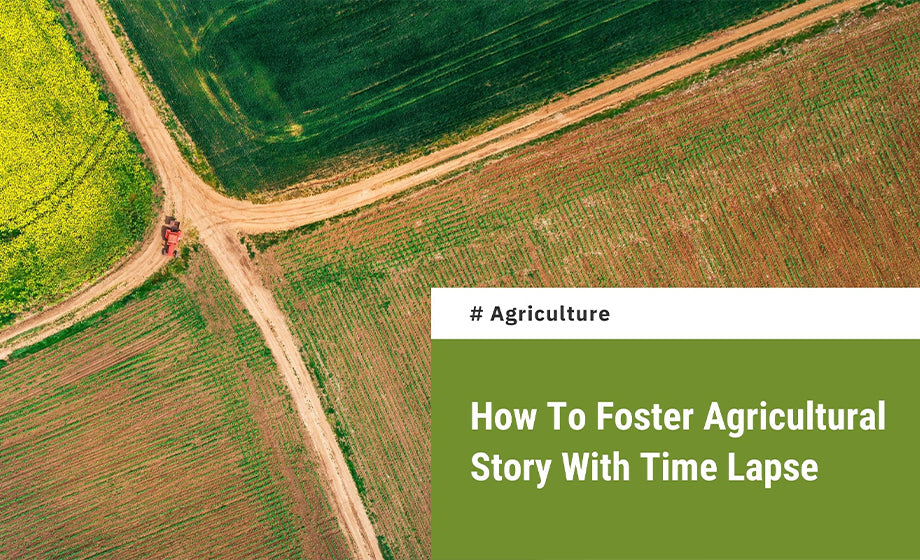The image is an overhead view of a patchwork of farm fields arranged geometrically. In the top left corner, a four-way intersection where dirt roads converge is visible. At this intersection, a small red tractor can be seen, though it's slightly obscured. The top left field is the smallest, with a yellowish-green hue and faint tire tracks across it. Adjacent to it, the top right field is a darker green, featuring several visible tire tracks. The bottom left and bottom right fields are primarily brown with intermittent green patches, suggesting recent seeding activity and early growth stages. Overlaying the lower right portion of the image is a text box. The top of this box has a white bar with the hashtag "agriculture" in black, while the remaining box area is olive green and contains white text that reads "How to foster agricultural story with time-lapse."